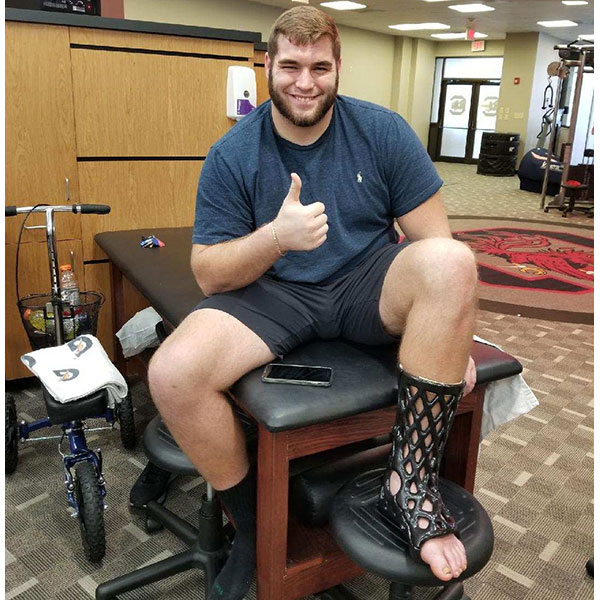This photograph captures a muscular man in his mid-20s, who is of Caucasian ethnicity with light brown hair and a beard, sitting on a physical therapy table. Dressed in gray shorts and a navy blue short-sleeve shirt with a polo logo, he faces the camera while giving a thumbs-up with his right hand. His left leg, adorned with a blue cast featuring mesh-like holes, is elevated on a stool. The professional setting, characterized by checked carpeting, French glass office doors, and an exit sign, suggests a modern, recent timeframe. In the room, various physical therapy equipment is visible, including a medical knee scooter with a Gatorade towel on its seat and Gatorade bottles in its front basket—one full of yellow Gatorade and the other empty. Behind him, exercise machines further indicate the clinical yet gym-like environment. He also has a phone resting in his lap, enhancing the contemporary feel of the scene.